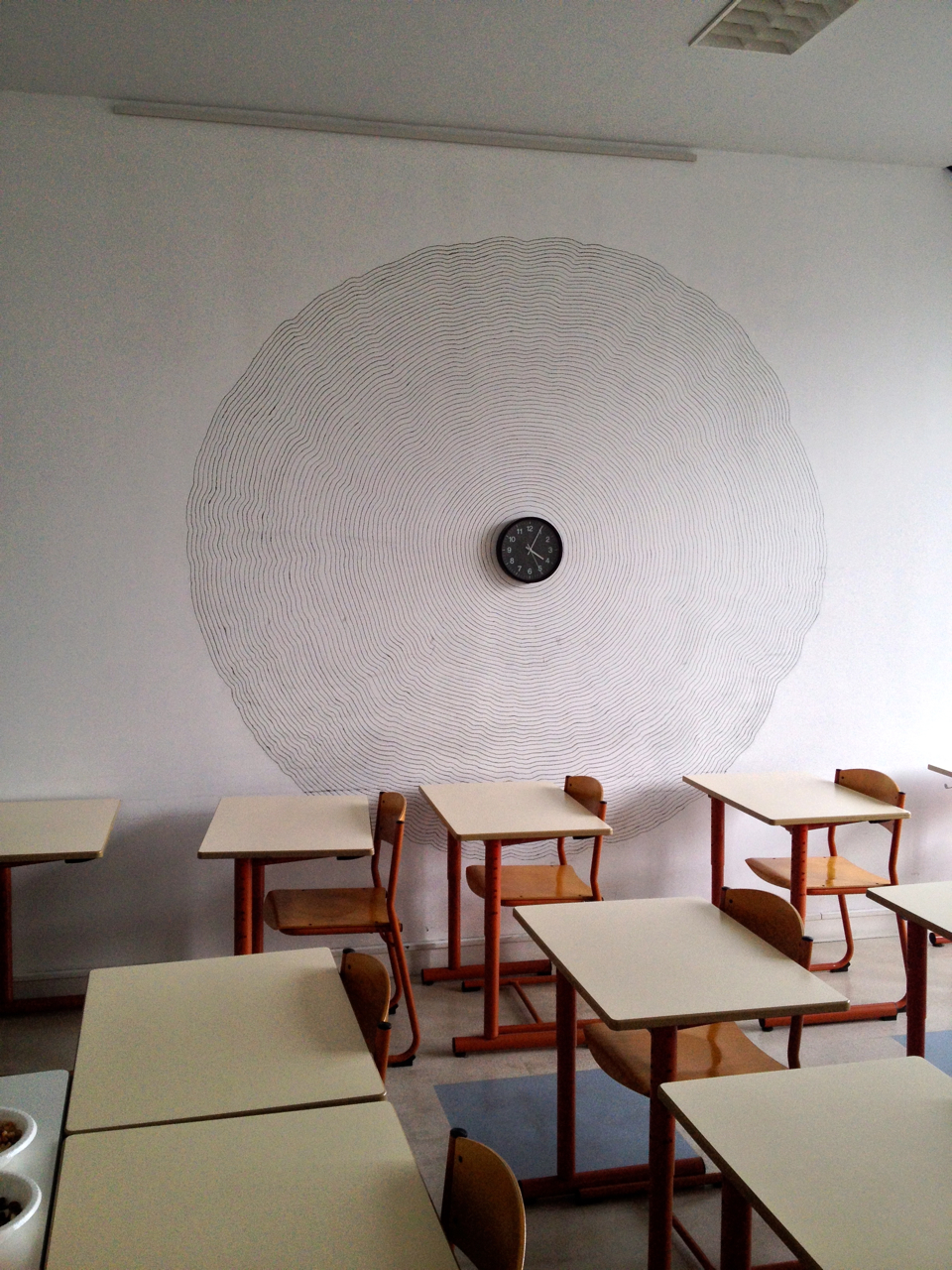The image depicts the interior of a school classroom, characterized by a series of white-topped, rectangular tables paired with plywood chairs. These chairs feature metal, tubular frames and are neatly positioned at each desk. The desks are arranged in slightly rotated vertical rows, approximately 30 degrees from the standard alignment. Dominating the far wall is an eye-catching design of large, black concentric circles set against a white background. At the center of this concentric design, a black clock with a matching black face and housing is prominently displayed. The clock's hands and numbers are in a golden-yellow hue, indicating the time as 4:05 PM.